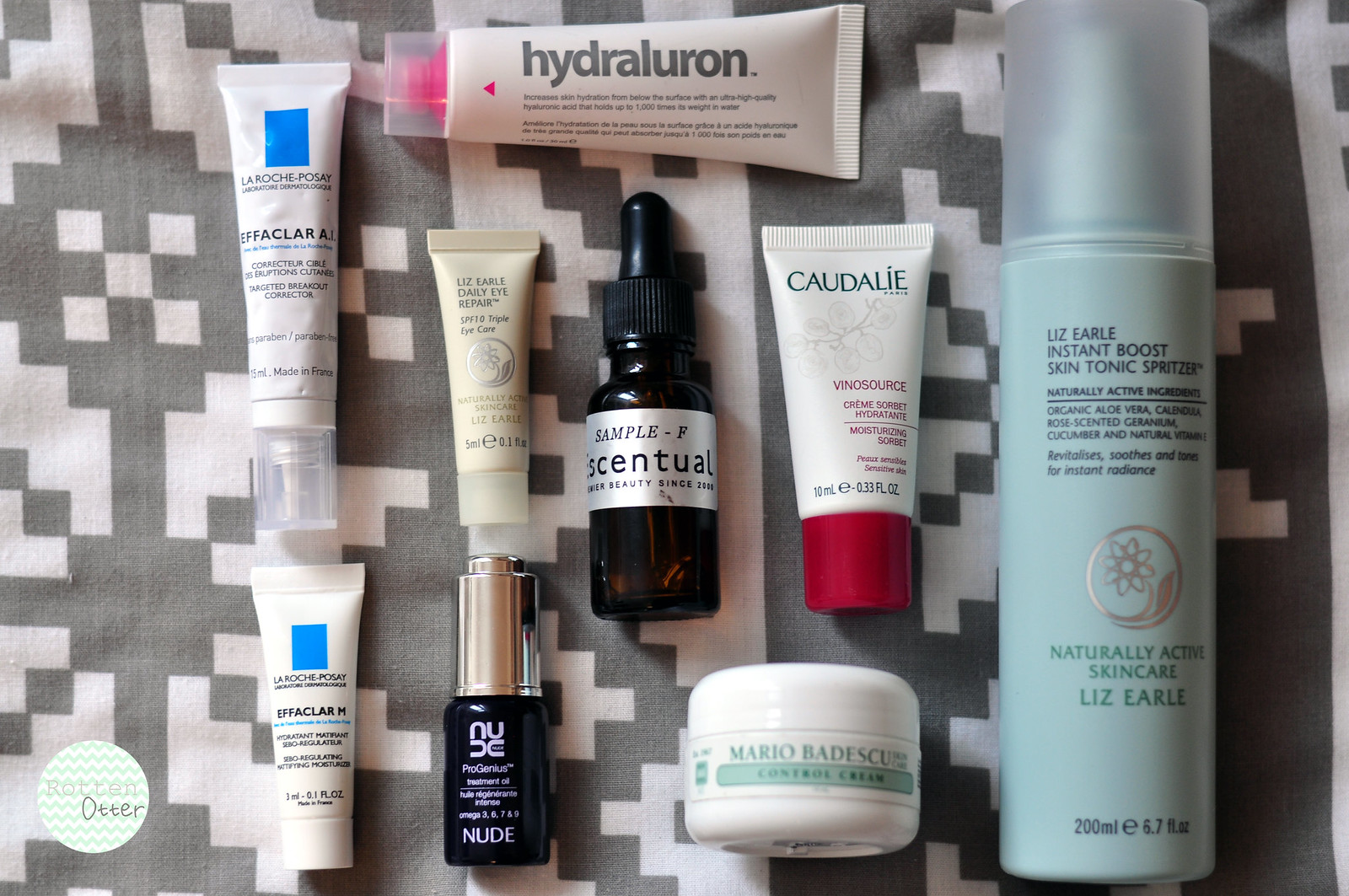A meticulously arranged collection of skincare products is displayed atop a soft cloth featuring a white backdrop adorned with intricate gray patterns reminiscent of vintage Atari video game block designs. The assortment includes various creams, serums, and lotions, each elegantly packaged, creating a visually appealing and harmonious composition against the retro-inspired fabric.